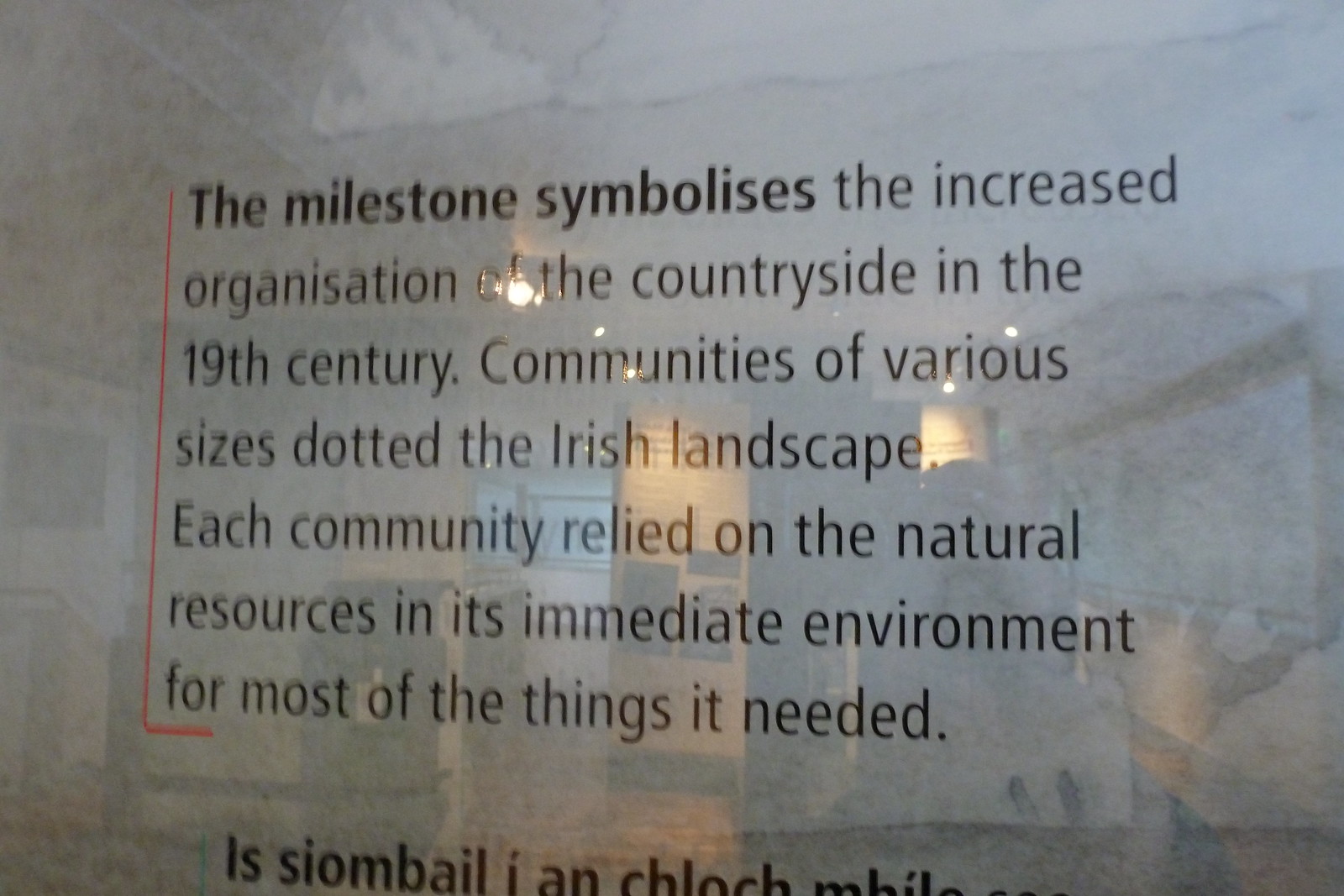The image features a reflective, shiny plaque mounted on what appears to be a marble surface, likely part of a museum exhibit. The plaque's black text is partially cut off at the bottom and reads: "The milestone symbolizes the increased organization of the countryside in the 19th century. Communities of various sizes dotted the Irish landscape. Each community relied on the natural resources and its immediate environment for most of the things it needed." The phrase "The milestone symbolizes" is emphasized in bold. The reflection in the plaque reveals a room with warm ceiling lights, and an L-shaped red line is visible to the left of the text, running along the side and bottom of the plaque, adding an artistic element. Some fragmented, likely non-English text appears at the bottom, indicating a multilingual display.